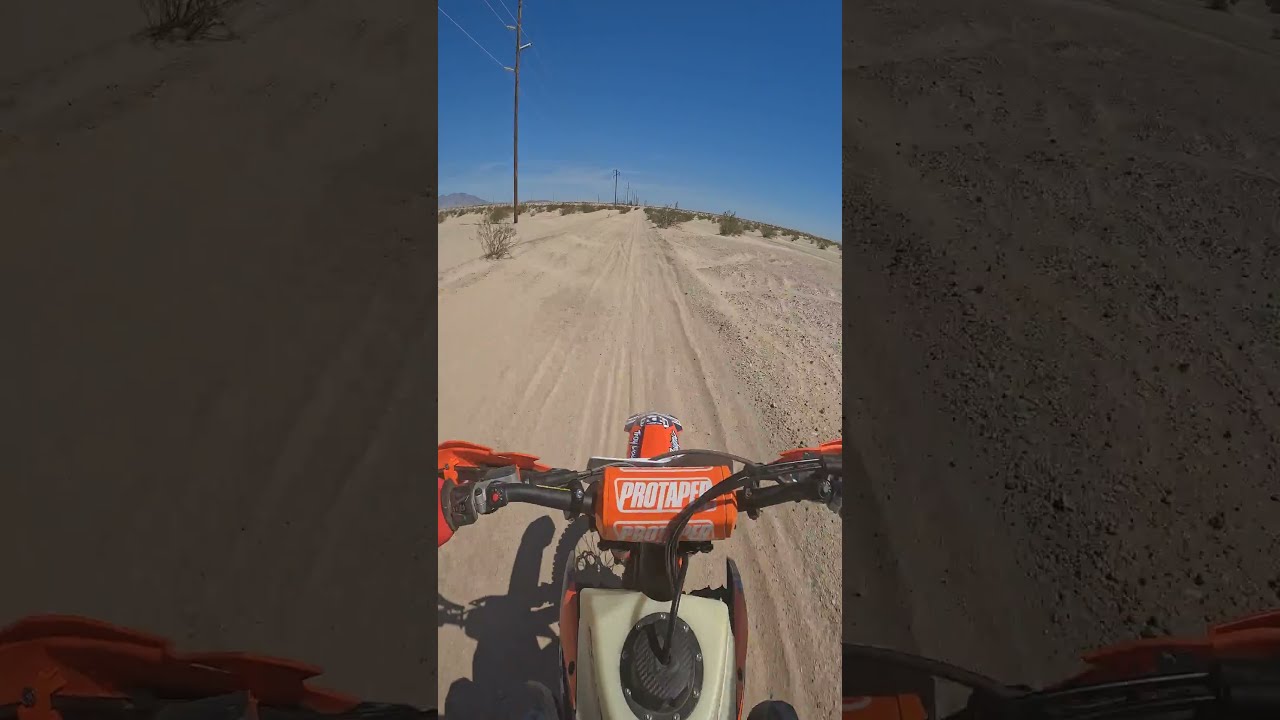This captivating image captures a close-up, first-person perspective of an individual riding an orange, black, and white dirt bike with the brand name "ProTaper" prominently displayed on the handlebar padding. The rider is navigating a desolate, desert-like terrain characterized by expanses of pale, sandy ground dotted with dry rocks, shrubs, sparse bushes, and occasional dry trees. The vast, empty landscape extends towards the horizon, void of any other people or vehicles. The sky above is a clear blue, accentuated by light, wispy clouds. In the distance to the left, a faint silhouette of a mountain can be seen, jutting into the expansive sky. The presence of telephone poles and electrical wires adds an industrial touch to this otherwise barren environment, emphasizing the remoteness of the location. The scene conveys a sense of solitary adventure, with the rider appearing to be on a swift, lonely journey through the seemingly endless desert.